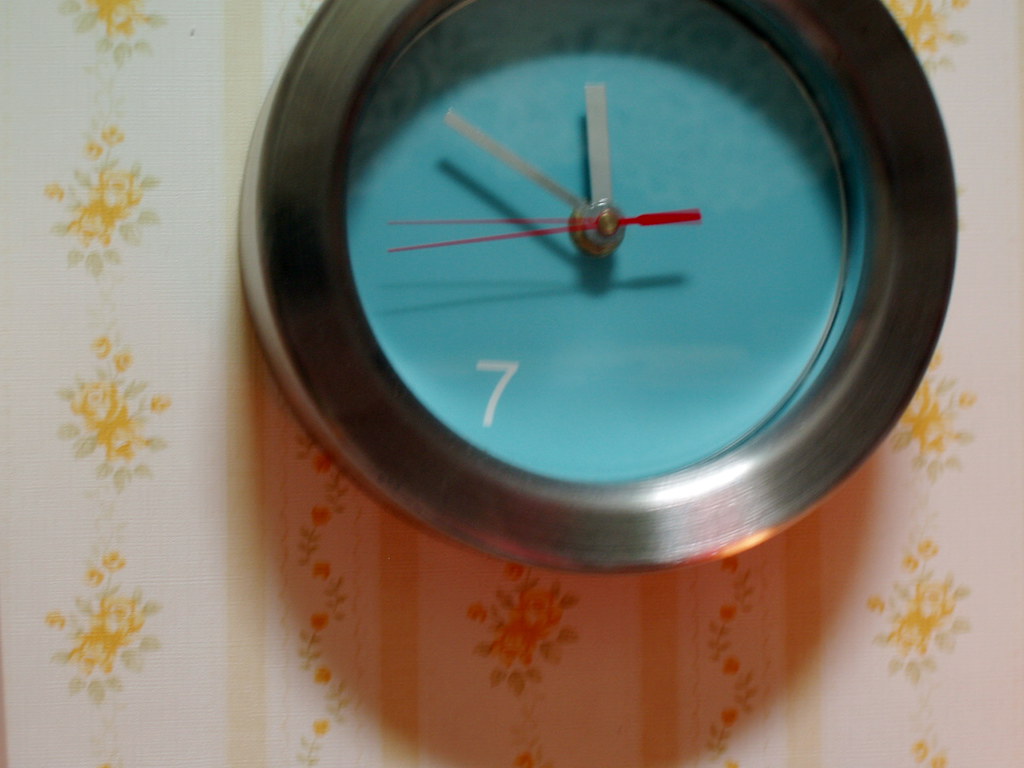This color photograph captures a rectangular image, slightly wider than it is tall, showcasing a round clock mounted on a wallpapered wall. The top of the clock is slightly clipped, revealing only most of its circular frame which is made of shiny metal, imparting a reflective border. The clock features a baby blue face with two sleek, silver metal hands indicating the hour and minute, and a red seconds hand. The time appears to be just before 12 o'clock. Notably, the only numeral present on the clock’s face is the number 7, positioned in the lower left quadrant and displayed in white. The backdrop is a wallpaper adorned with yellow flowers and light beige vertical columns, which add an element of vintage charm to the setting.